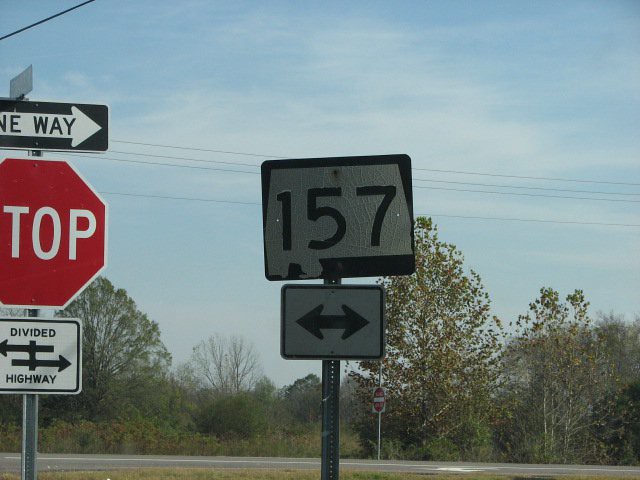In this image, there are multiple street signs situated at the side of an asphalt road adorned with white lines. On the left side of the image, there is a black and white 'One Way' sign featuring an arrow pointing to the right. Just below it, a red and white 'Stop' sign is visible, alongside a black and white 'Divided Highway' sign indicating the beginning or continuation of such a road.

Towards the right of the image, a black and white sign displays the number '157.' Positioned directly beneath it is another black and white sign featuring arrows pointing both left and right, suggesting direction options.

In the background, there are green trees under a blue sky scattered with thin white clouds. Additionally, a distant sign across the street shows a white and red 'Do Not Enter' symbol.